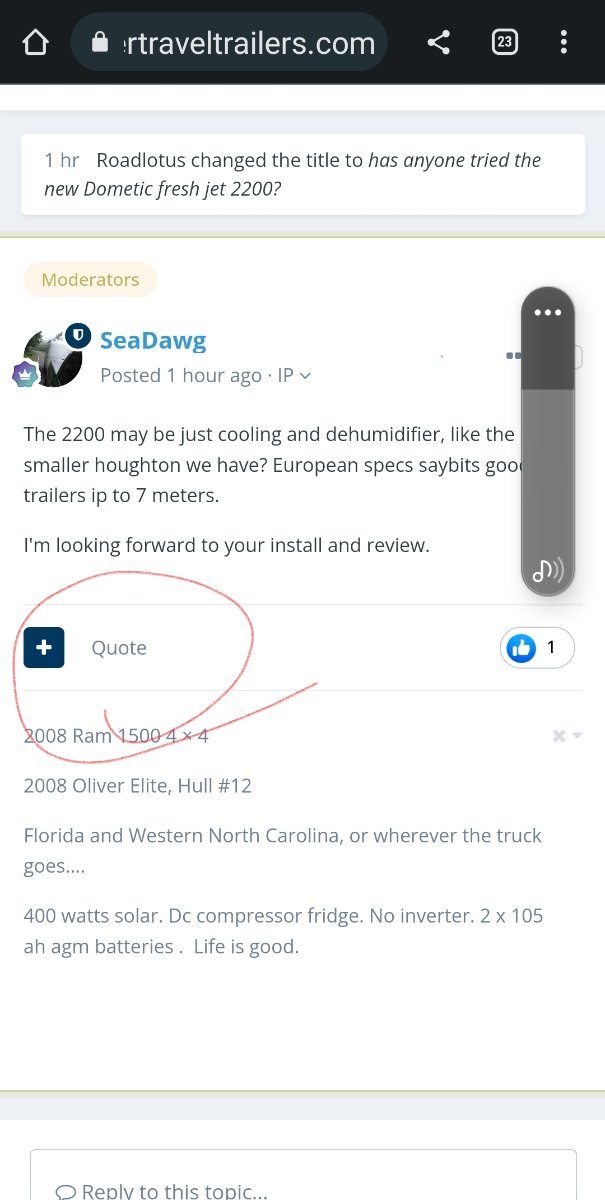The image is a detailed screenshot of someone's cell phone displaying a webpage. At the top, on the black navigational bar, there's a house icon for the home button on the left. Adjacent to it, partially visible in the search bar, is a URL segment "rtraveltrailers.com." This is followed by a share symbol, a "23" in a square, and three vertical dots at the far right. Below the bar, in grey font, the timestamp "1 hour" is displayed, while the title "Road Lotus" appears next to it in black. The title is suggested to be revised to "Has Anyone Tried the New Dometic Fresh Jet 2200?" set against a white background.

Further down, on another white background, there's a label "Moderators" situated in an elongated light pink oval. The word "Moderators" is in a yellowish hue, accompanied by a crown symbol on the left and a shield symbol above a circular avatar on the right. The user, Seadog, whose name is displayed in blue, posted this 1 hour ago. Their post reads: "The 2200 may be just cooling and a dehumidifier like the smaller Houghton we have. European specs say it's good trailers IP to 7 meters. I'm looking forward to your install and review."

A volume symbol indicating high volume appears in a light grey and dark grey box with three horizontal dots. Below is a large red circle containing a plus sign, next to which is a quote icon. Across from the quote icon is a blue circle with a white thumbs up, accompanied by the number 1. The text beneath the quote describes: "2008 Ram 1500 4x4, 2008 Oliver Elite, Hull 12, Florida and Western North Carolina or wherever the truck goes... 400 watt solar. DC compressor fridge. No inverter. 2x105 AH AGM batteries. Life is good." 

At the very bottom, another light grey rectangle contains the text "reply to this topic."